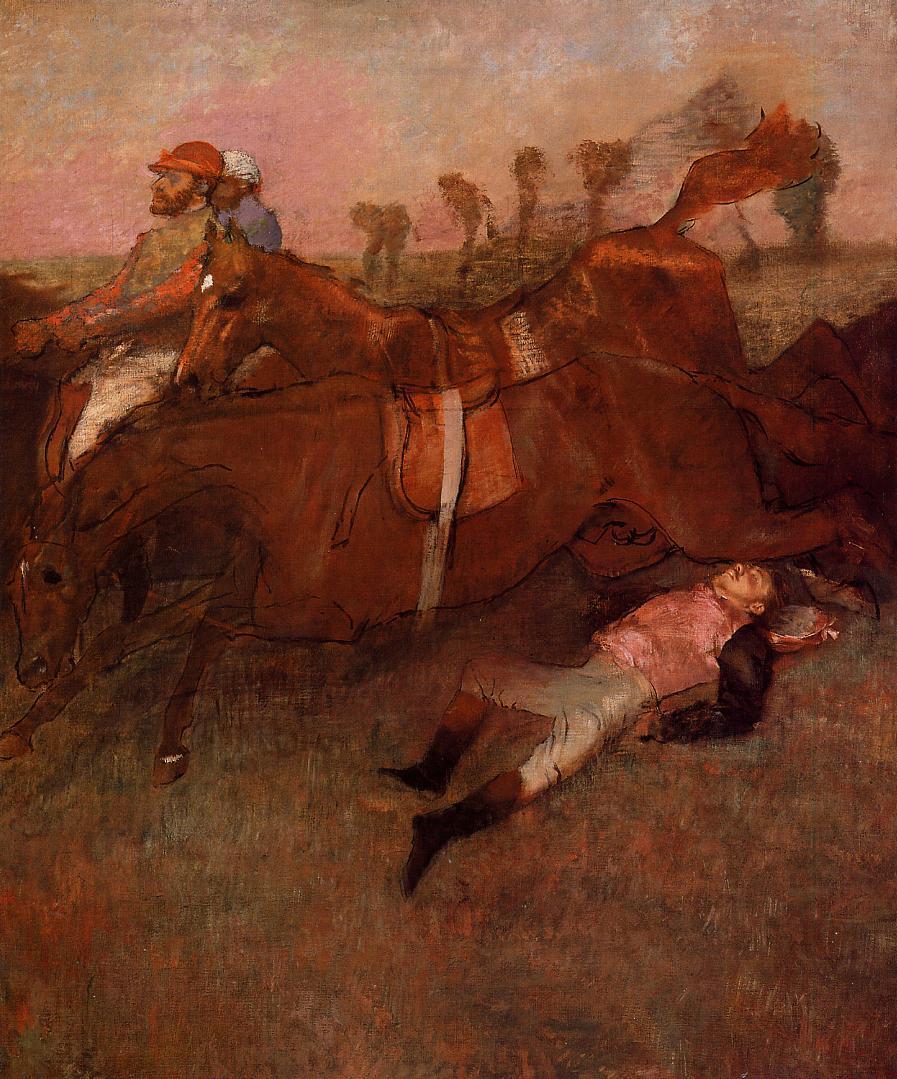This dynamic painting depicts a dramatic horse race scene captured in a vivid artistic style. The background features delicately rendered silhouettes of palm trees against a softly blotched sky of pink, blue, and brown hues, indicating a daytime setting. In the foreground, two brown horses with red saddles are shown in mid-leap, their side profiles pointing to the left, seemingly jumping over a fallen jockey. This unfortunate man, possibly unconscious, lies on the ground with his eyes closed. He wears black boots, white riding pants, and a pink shirt with black sleeves, suggesting he might have been knocked out from his fall. His legs are sprawled beneath one of the horses near the bottom right of the painting. 

Two visible jockeys are still mounted on their horses in the background. The jockey on the left, adorned with an orange riding helmet and matching shirt with white pants, sports a distinctive full red beard. The jockey on the right, in a white helmet and blue shirt, has his lower body obscured by his horse's head. Both jockeys are of Caucasian descent and give a sense of urgency and competition to the scene as their horses charge forward. The overall impression is one of motion and tension, capturing a fleeting moment in the heat of a race.